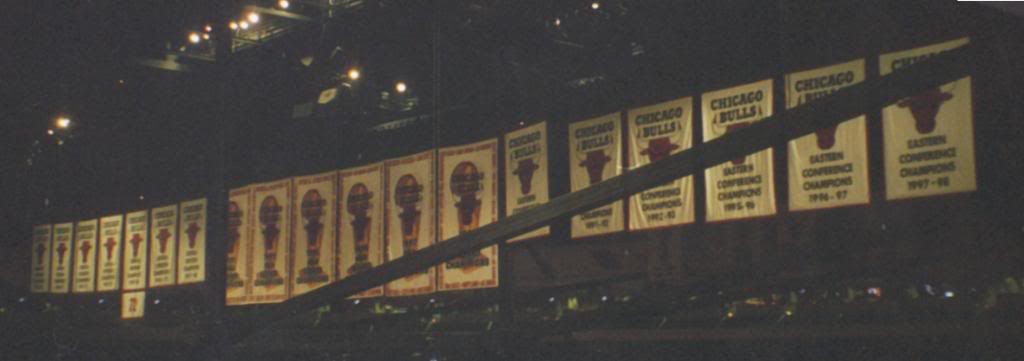This panoramic image showcases a dimly lit arena adorned with numerous championship banners and team flags. Starting from the right, there are six prominent banners for the Chicago Bulls, each with the team's name boldly displayed at the top in black letters against a white backdrop, accompanied by the iconic red bull's head with horns. Some banners are legible; for instance, the rightmost banner touts the Bulls as Eastern Conference Champions for the 1997-98 season, with the adjacent banner celebrating the 1996-97 season. 

Moving leftward, four more Bulls banners are visible, followed by six banners for another basketball team, and then an additional set of Bulls banners. Dominating the image are the bright lights positioned at the top, signaling the arena’s rafter, though the overall scene remains largely dark, suggesting low ambient lighting or a filter effect. Despite some architectural structures partially obscuring the view, the presence of multiple Chicago Bulls banners, along with the championship insignias, clearly identifies this as a stadium, likely during a moment of stillness and reverence for the team's illustrious history.